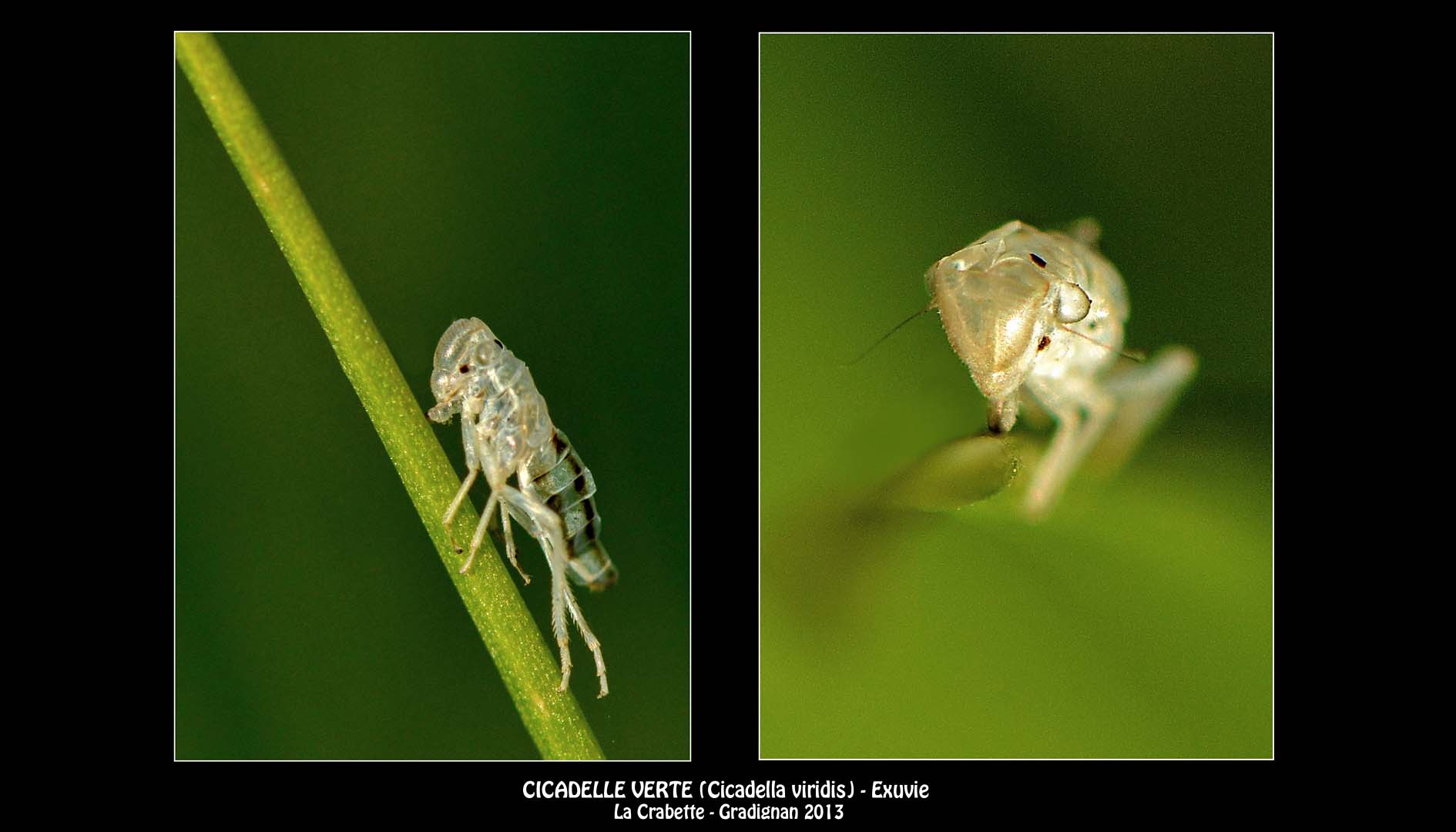The image consists of two photographs of an insect displayed on a black background, each bordered by thin gray lines. On the left, the insect, which is a translucent light green with green and yellow hues, is seen from the side as it climbs a slender green stem. The insect's three visible legs on this side grip the stem, and it has a noticeable eye and a striped tail. The background behind this photograph is a blurry green, giving a sense of depth. On the right, a head-on view of the insect reveals its triangular-shaped head and intricate details in green and gold against a similarly blurred green backdrop. Below the right photograph, in white capital letters, is the text "Cicadelli Verte," followed by the name and details of the print, "La Crabbit - Gradignon 2013," credited to the photographer Kaikadel Veritas exuvi.